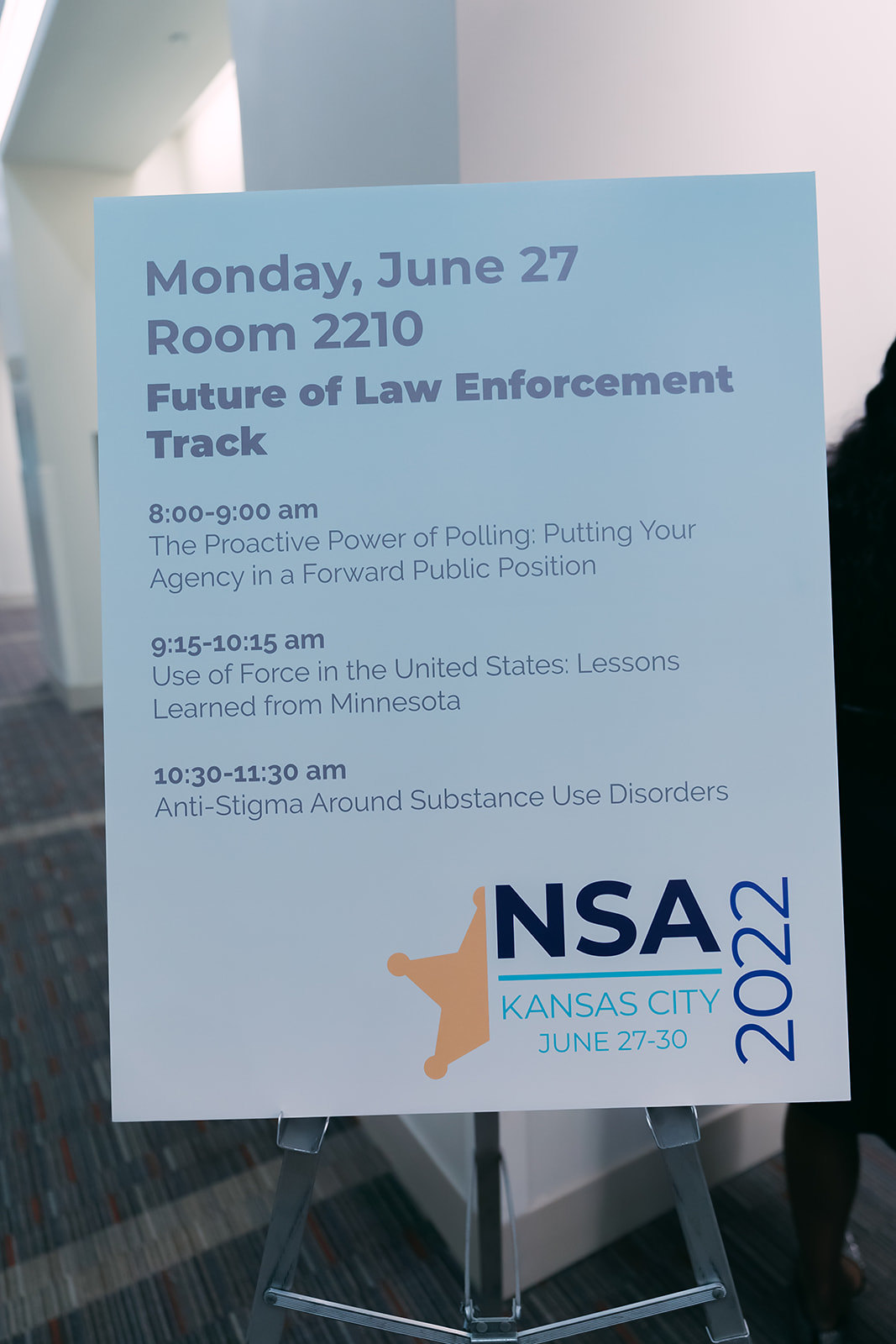The image features a light blue sign mounted on a silver tripod stand positioned on a striped carpet with hues of red and blue, against a backdrop of white walls. The sign details the agenda for a seminar slated for Monday, June 27th, in room 2210, under the theme "Future of Law Enforcement Track." The itinerary begins with "The Proactive Power of Polling: Putting Your Agency in a Forward Public Position" from 8:00 to 9:00 a.m., followed by "Use of Force in the United States: Lessons Learned from Minnesota" from 9:15 to 10:15 a.m., and concludes with "Anti-Stigma Around Substance Use Disorders" from 10:30 to 11:30 a.m. At the bottom of the sign, in black text, it reads "NSA 2022" with a gold sheriff's star to the left, and below it "Kansas City, June 27 to 30." There is also a person visible in the background on the right side behind the sign.